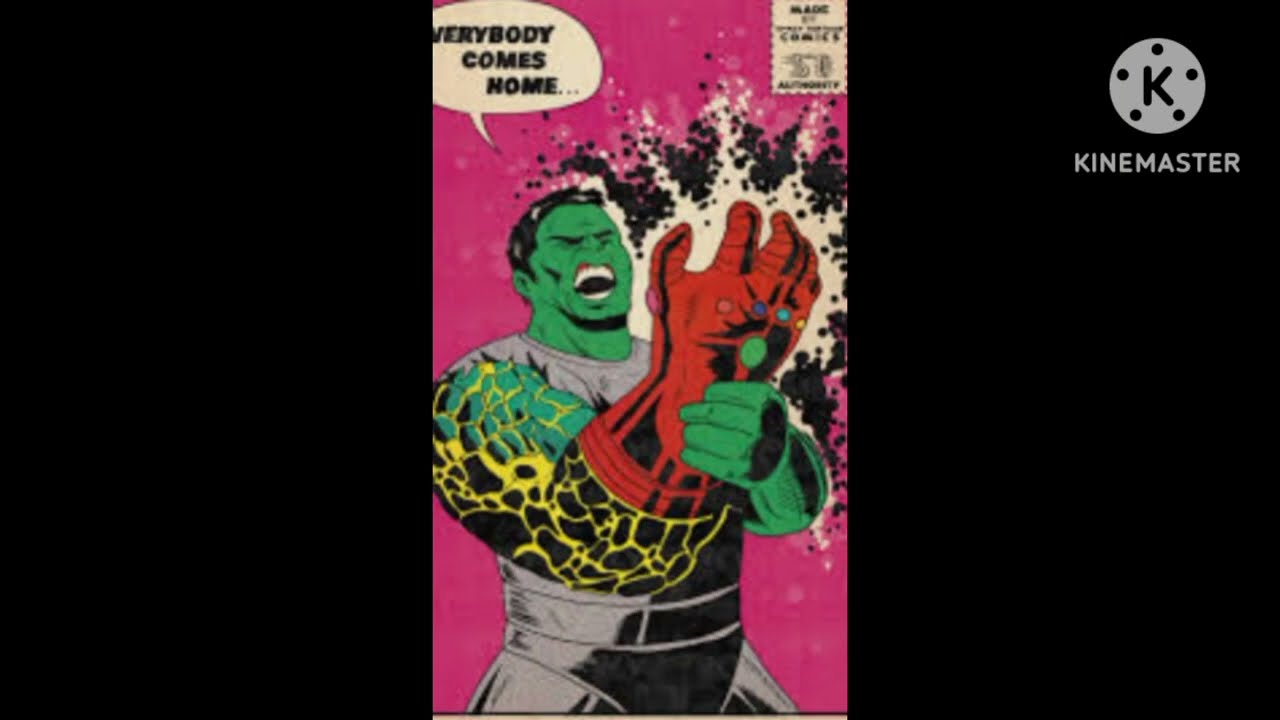The image features a vibrant comic book cover set against a large black background, with the borders on the left and right sides. In the top right corner of this black backdrop, there's a white circle containing a black 'K', beneath which "KineMaster" is written. The central, vertically-oriented image is dominated by a bright pink background and showcases a character resembling the Incredible Hulk. The Hulk-like figure appears to be in immense pain, his facial expression contorted with his mouth open as if yelling. He wears a red glove on his left hand, reminiscent of the Infinity Gauntlet, which is emanating intense bursts of black and white energy. The left arm of the character looks swollen and cracked, glowing with yellow light. A white speech bubble with black text near his head reads, "Everybody comes home..." In the upper left corner of the image, there is a comic stamp that reads "Something Made Comics" along with a price.